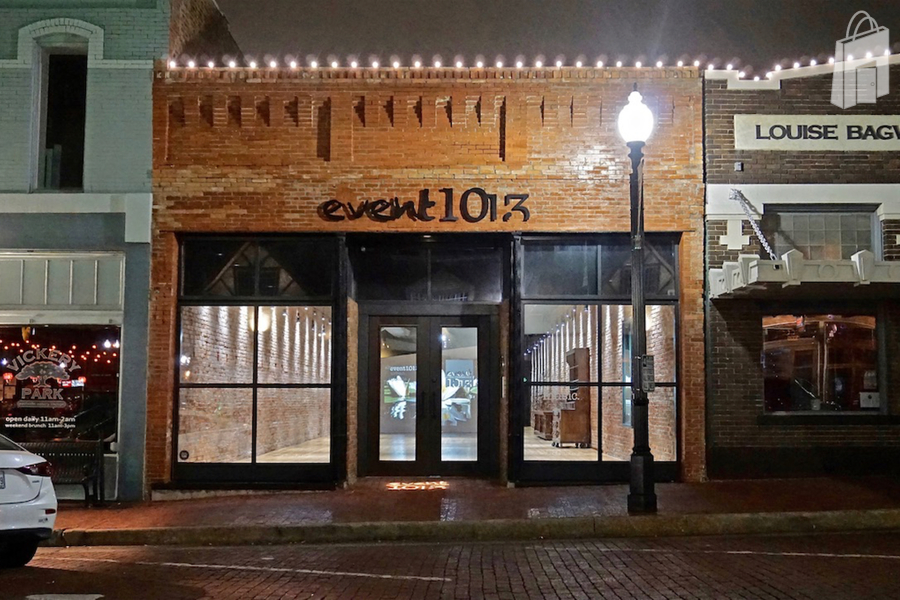This nighttime photograph captures a charming city street with cobblestone surfaces, including both the sidewalk and the road, which shimmer as if wet from a recent rain. The scene prominently features a brown brick building with black trim, identified as Event 1013, situated in the center. This storefront boasts double doors flanked by four square windows on either side, all highlighted by a well-lit streetlight that enhances the visibility of the building’s distinctive black edging and trim. The ground-level signage reads "Event 1013," with small windows forming large squares around the entrance, hinting possibly at an antique or furniture store given the visible desk and hutch inside.

Adjacent to Event 1013, the storefront on the right is darker, partly obscured by an overhanging awning. The sign reads "Louise BAG" with an unreadable final letter, creating an intriguing mystery. On the left, another storefront, identified as Vickery Park, has its name painted on a large window. The scene is completed with the partial view of a white car parked alongside the road, further emphasizing the quaint yet lively urban atmosphere.